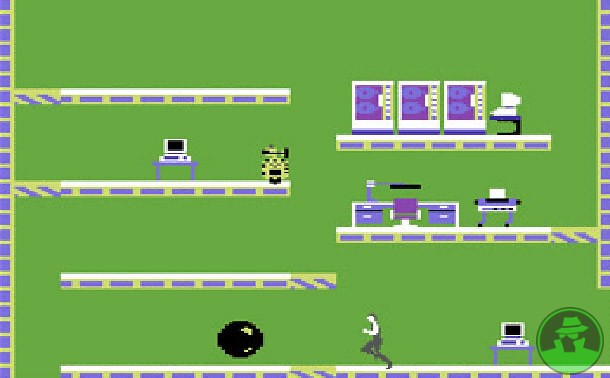The image is a detailed screenshot from an old-school, platform-style video game, possibly from the era of Atari or early Nintendo, reminiscent of early 80s graphics. The entire background is green with various shades giving it a medium green hue. Four distinct levels or platforms, which are colored in purple and yellow, form the structure of the game. These are designed to be climbed by the player's avatar, who is positioned at the bottom of the screen. The levels contain various animated elements, including little computers and desks as well as other machinery. On the top platforms, additional machinery and animated objects can be seen, such as a plant on a desk. The player’s character appears to be running towards or away from a large black object, which could be interpreted as a bowling ball or a bomb. Each platform has a meticulous design with green dashes and purple lines or squares that run down both sides, adding to the nostalgic aesthetic of the game.